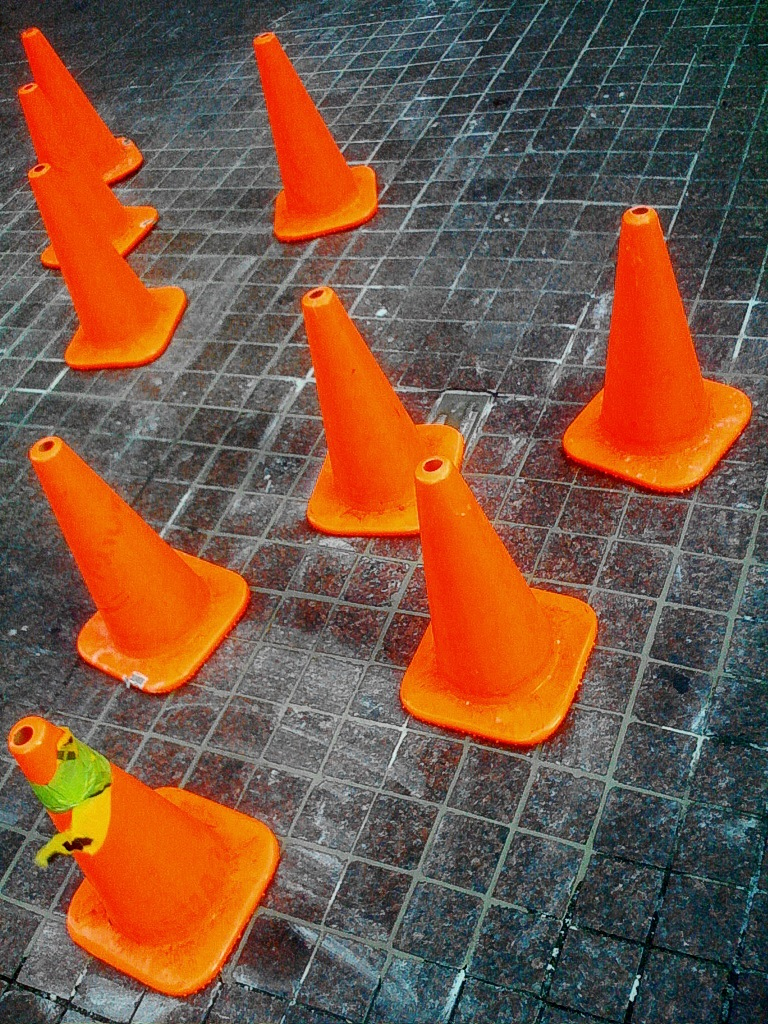The image features nine short orange traffic cones, approximately a foot and a half tall with a six-by-six-inch base, scattered haphazardly across a walkway composed of dark, multicolored tiles. The tiles appear to be either dark black or dark blue, punctuated by light green or gray grout, which is missing in some places. The floor seems to have been recently cleaned but still shows a white residue scattered around the cones, hinting at ongoing construction or other maintenance work. Notably, one cone in the bottom left corner bears a torn piece of caution tape and a plastic sticker near the top, colored yellow and green. The overall scene is devoid of people, focusing solely on the seemingly random placement of the cones amidst the mixed-colored tiling.